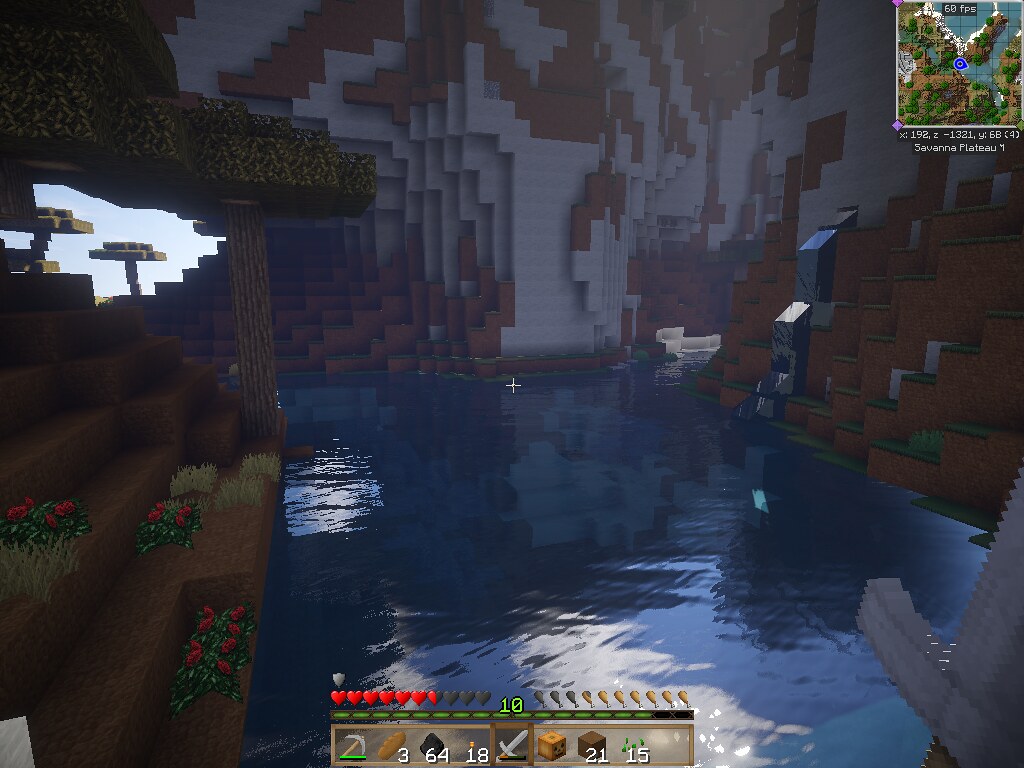This is a detailed screenshot from the video game Minecraft. The central focus of the image is a blue river with reflections of white ripples, indicating movement. On the left side, adjacent to the river, are brown stairs descending off the edge of the frame. Surrounding these stairs are green patches of grass, red flowers, and leaves. Further to the left, there is a garden area with trees. The terrain is constructed in the characteristic block style of Minecraft. On the right, a white concrete wall adorned with brown and red-brown patterns leads into the scene, featuring interconnecting square designs. Gray and brown blocks line the pathway on the right side of the river. In the lower right corner, the hilt of a gray sword is visible, suggesting the player is armed. The player's inventory is displayed at the bottom center of the screen, featuring several icons that denote materials and the player’s current health status, indicated by hearts that are both red and gray. The top right corner of the image contains a map showing the player's position in the game world.